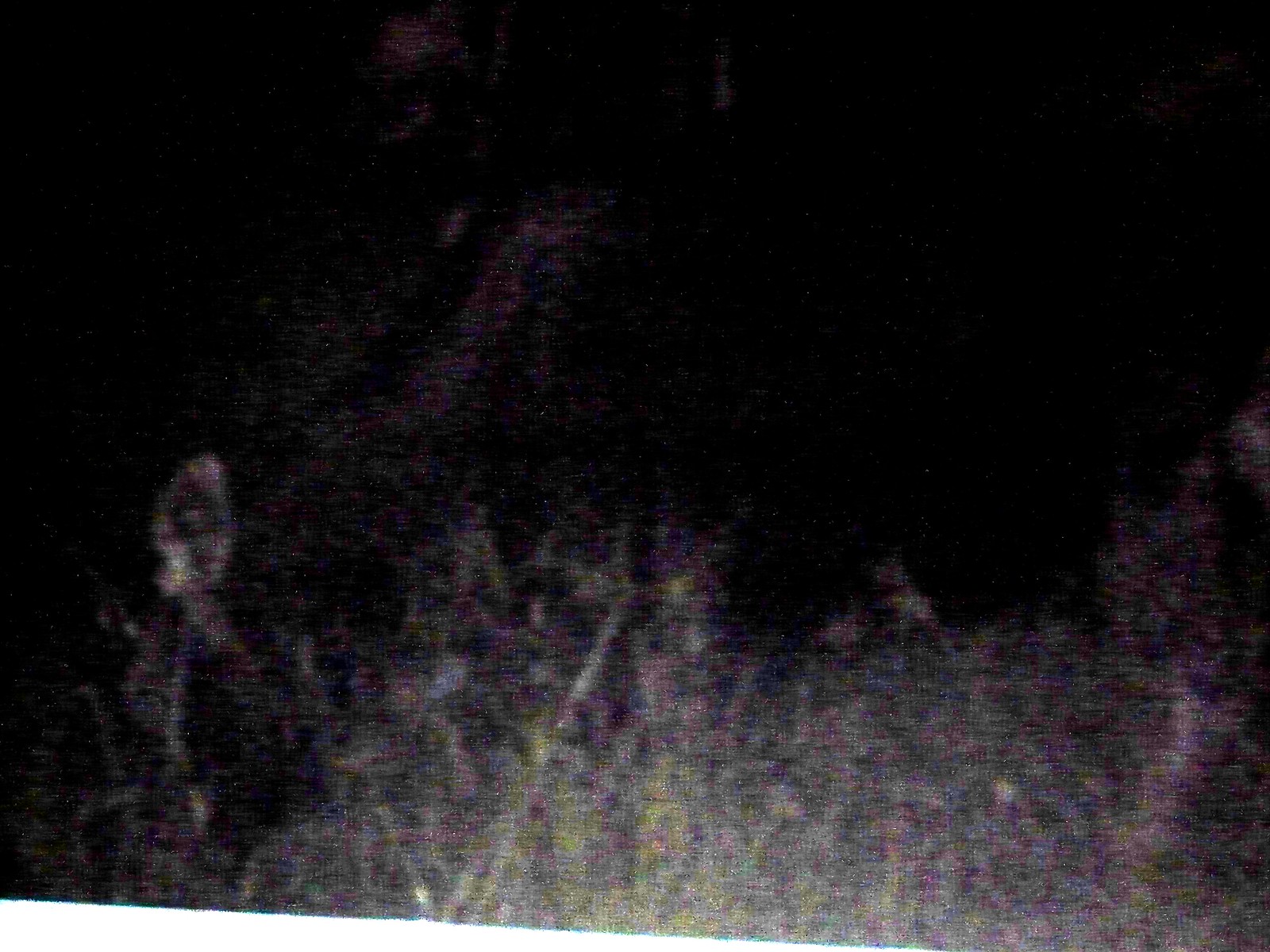A dimly lit outdoor photograph predominantly shrouded in darkness. The upper two-thirds of the image is almost entirely black, suggesting it was taken at night or in very low light conditions. The bottom portion reveals a faintly illuminated patch, apparently touched by some light source, depicting a variety of plants. These plants display a mix of green, yellow, and purplish-pink hues, giving the impression of weeds, grass, or wildflowers. On the left side of the image, an indistinct object stands out, its shape vaguely reminiscent of a hangman figure, characterized by a thin stalk and some ambiguous appendages. The overall image is blurry and lacks proper lighting, making it difficult to discern specific details and leaving much to the viewer's imagination.